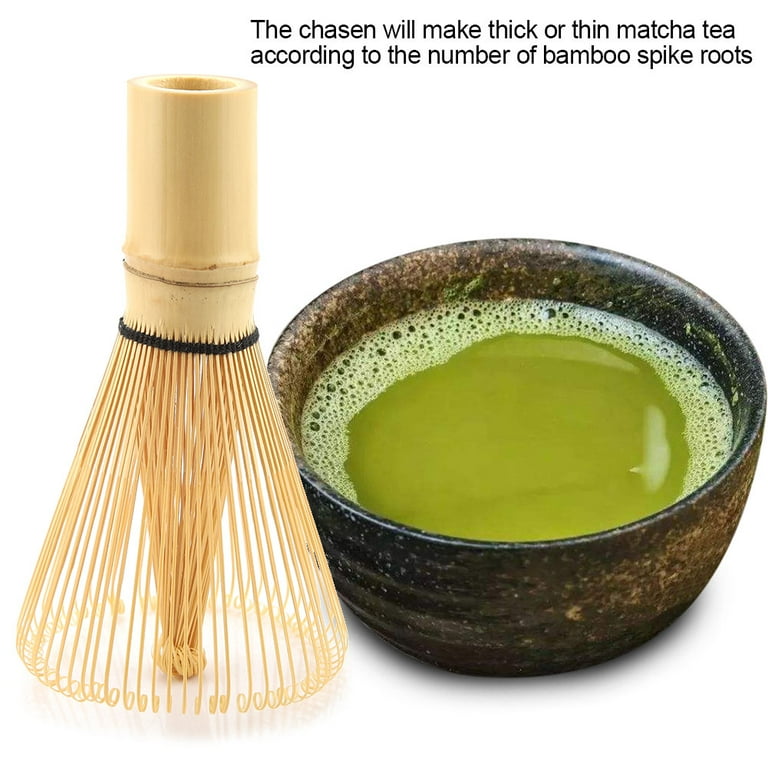This image shows a detailed setup for preparing matcha tea against a white background. Central to the image is a small, dark stoneware bowl, which features a deep, earthy color palette—a mix of brown and black speckles, giving it a natural and rustic appearance. The bowl is filled with a light, translucent green liquid, characteristic of matcha tea, with bubbles forming a ring around the rim. Adjacent to the bowl is a traditional bamboo whisk known as a chasen. The chasen is crafted from a single bamboo stalk, meticulously cut into numerous fine, thin strips that fan out in a cone shape and curl at the ends. A black band around the base binds the strips together. Above the bowl is a textual description that states, "The chasen will make thick or thin matcha tea according to the number of bamboo spike roots," indicating the whisk's function in mixing the matcha to the desired consistency.